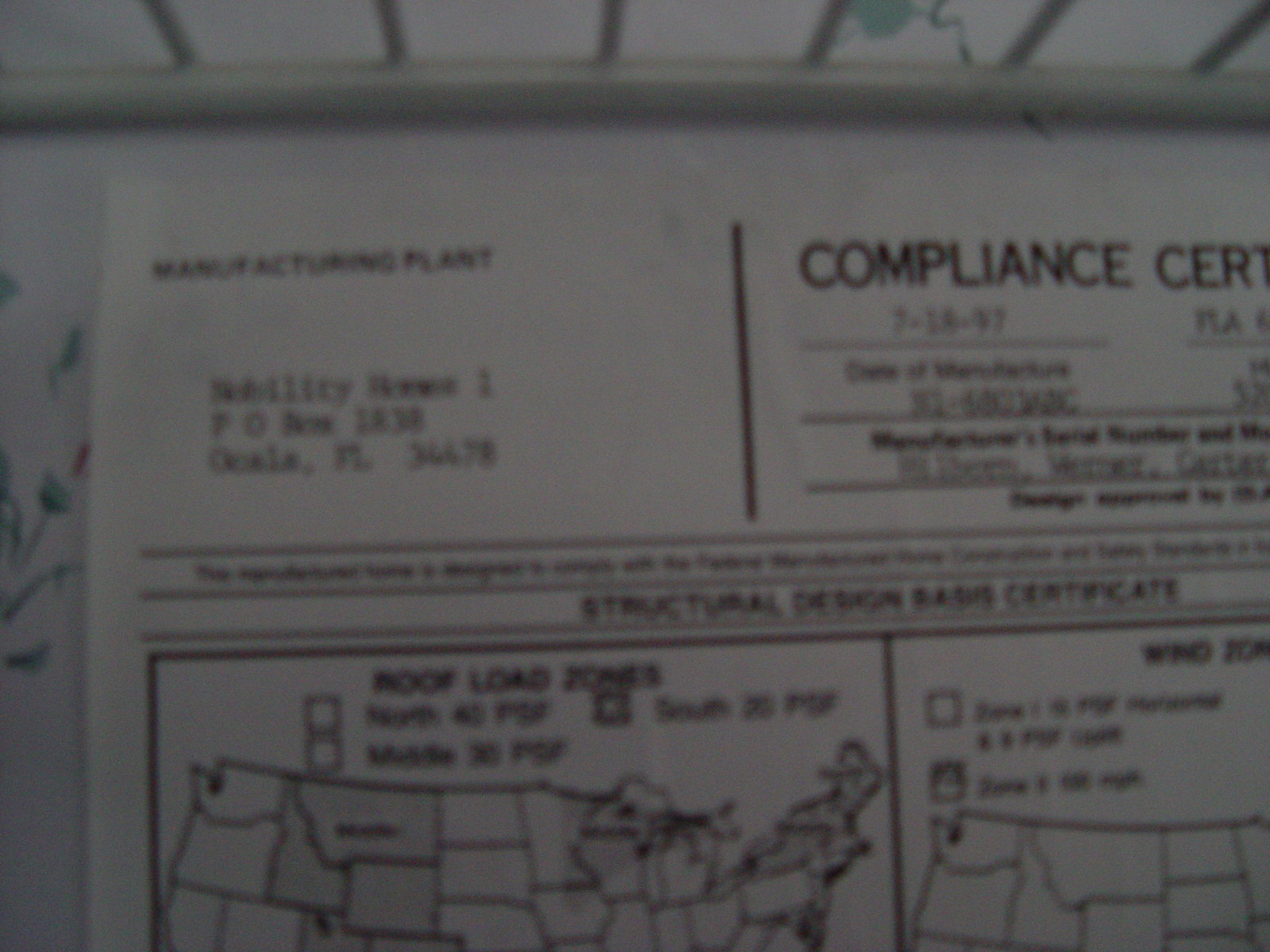In this slightly blurred image, a piece of paper, likely a compliance certificate, is prominently featured. The top of this document displays the words "Compliance Cert" in bold, though the rest of the text is unclear due to the image quality. On the top left, there's an address with mention of a P.O. Box in Ocala, Florida, including a zip code that is not legible. Below this, there is a section with the term "Structural" followed by indecipherable text, ending with the word "Certificate." In the lower portion of the paper, there are two maps of the United States, one labeled "load zones," with additional unreadable text above them. The background of the image includes a wall adorned with vertical whiteboards and lightly painted flowers in hues of blue, green, and red on the left side, as well as part of a ceiling. The exact positioning of the paper—whether it's on a table or against the wall—remains ambiguous. The overall document appears to relate to structural planning or compliance in black and white.